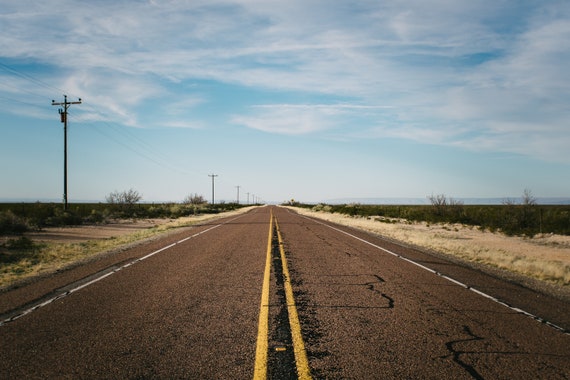The image depicts a very rural, desolate highway stretching into the distance, characterized by weathered black and gray asphalt. The faint double yellow lines run steadily through the middle of the road, emphasizing its seeming infinity. The pavement is grainy with pebbles and is marked by numerous cracks that have been filled with black tar. Flanking the road on either side are barren shoulders of dry, brownish grass, interspersed with sparse bushes and leafless trees. To the left, a line of telephone poles recedes into the background, echoing the road’s endless stretch. The scene is capped by a pale blue sky scattered with wispy, hazy white clouds, creating a serene yet isolated atmosphere. There are no vehicles, no traffic—just the empty, silent road cutting through a quiet landscape.